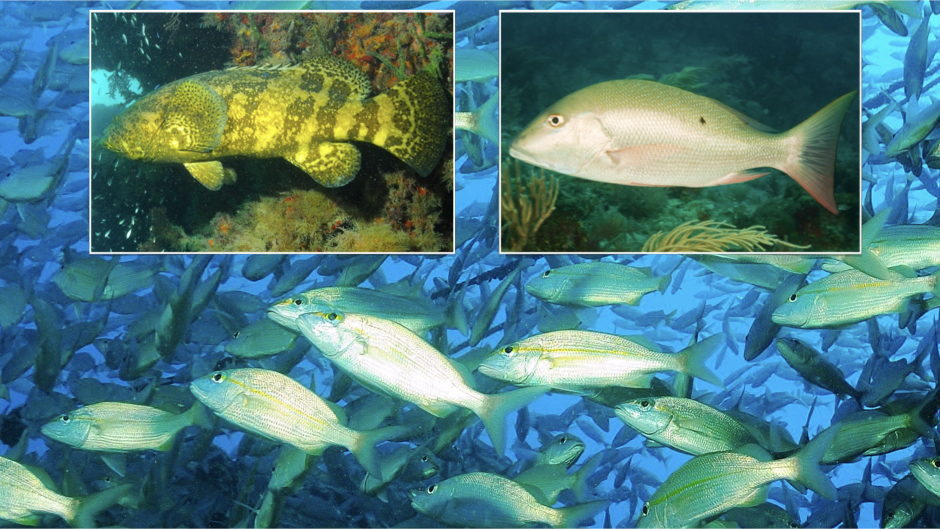This detailed illustration features a vibrant underwater scene set in a blue ocean. The primary background showcases a large school of shiny silver fish with yellow markings and eyes, numbering in the hundreds or even thousands, all swimming towards the left. Ocean vegetation, depicted with medium-sized, bush-like leaves, adds depth to the aquatic environment. 

In the upper portion of the image, two close-up insets of different fish are prominently displayed. The left inset features a yellow and brown fish with fan-shaped tail and blackish stripes, swimming amidst ocean plant life. This fish’s eyes are less visible, perhaps due to the angle or detail of the illustration. 

The inset on the right presents a fish similar to those in the background school, with a silver bottom half and a yellowy-green top. This fish is distinguished by its gold-colored eye, a small black spot on its back, and a salmon-colored accent line under its back fin and along one of its gills. Together, these elements create a rich, detailed portrayal of marine life.